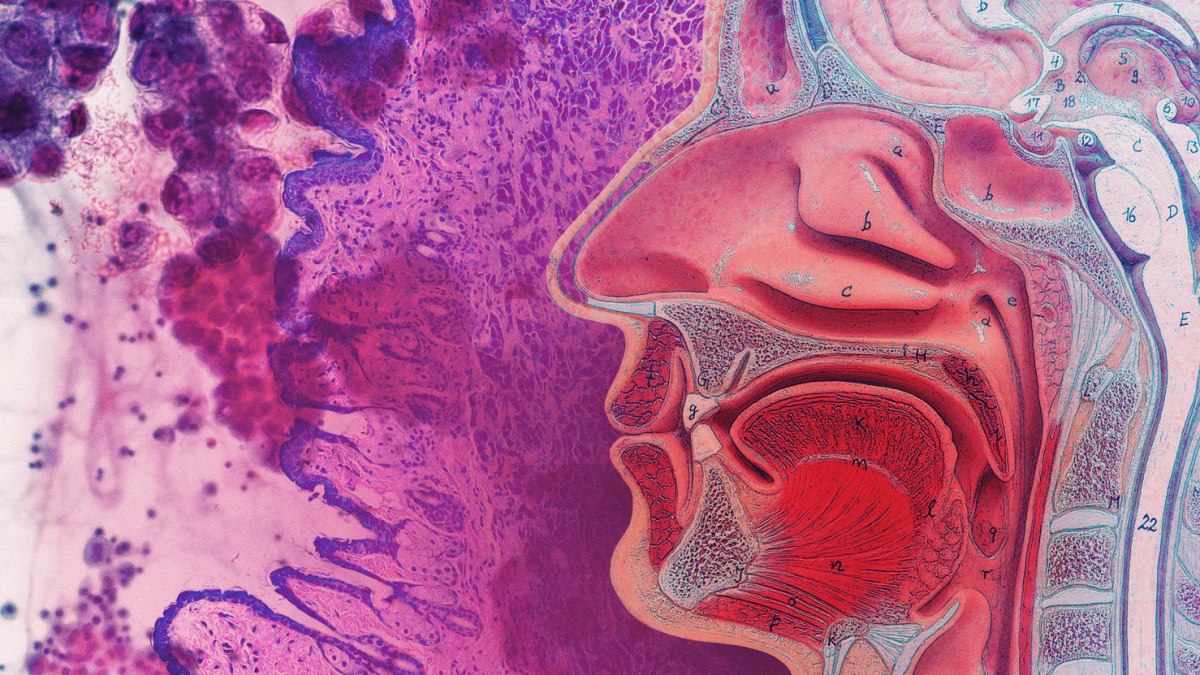The image presents an intriguing fusion of scientific accuracy and artistic expression. On the right side, it features a detailed, cross-sectional profile of a human face, reminiscent of anatomical textbook illustrations. This profile showcases the skeletal and muscular systems prominently, with clearly labeled parts including the lips, sinus cavities, tongue, uvula, nasal passages, and the spinal column. Each anatomical section is marked with a combination of letters and numbers (e.g., A, B, C, D, 11, 17), suggesting the presence of an accompanying key. The image cuts off just above the eyes and extends down to include the base of the brain and the upper portion of the spinal cord.

The left side contrasts sharply with an abstract, purplish background that resembles a wash of watercolors, featuring splotches and splashes of varying shades of purple, pink, and red-violet. This side evokes a more fluid, organic feel, dotted with shapes that could be interpreted as cells or microscopic elements, enhancing the sense of a histological study. The overall aesthetic is both educational and evocative, suitable for the cover of a medical or scientific publication, with its blend of structured anatomical detail and freeform artistic design. The ambiguous gender of the profile adds to the universal appeal and scientific neutrality of the piece.